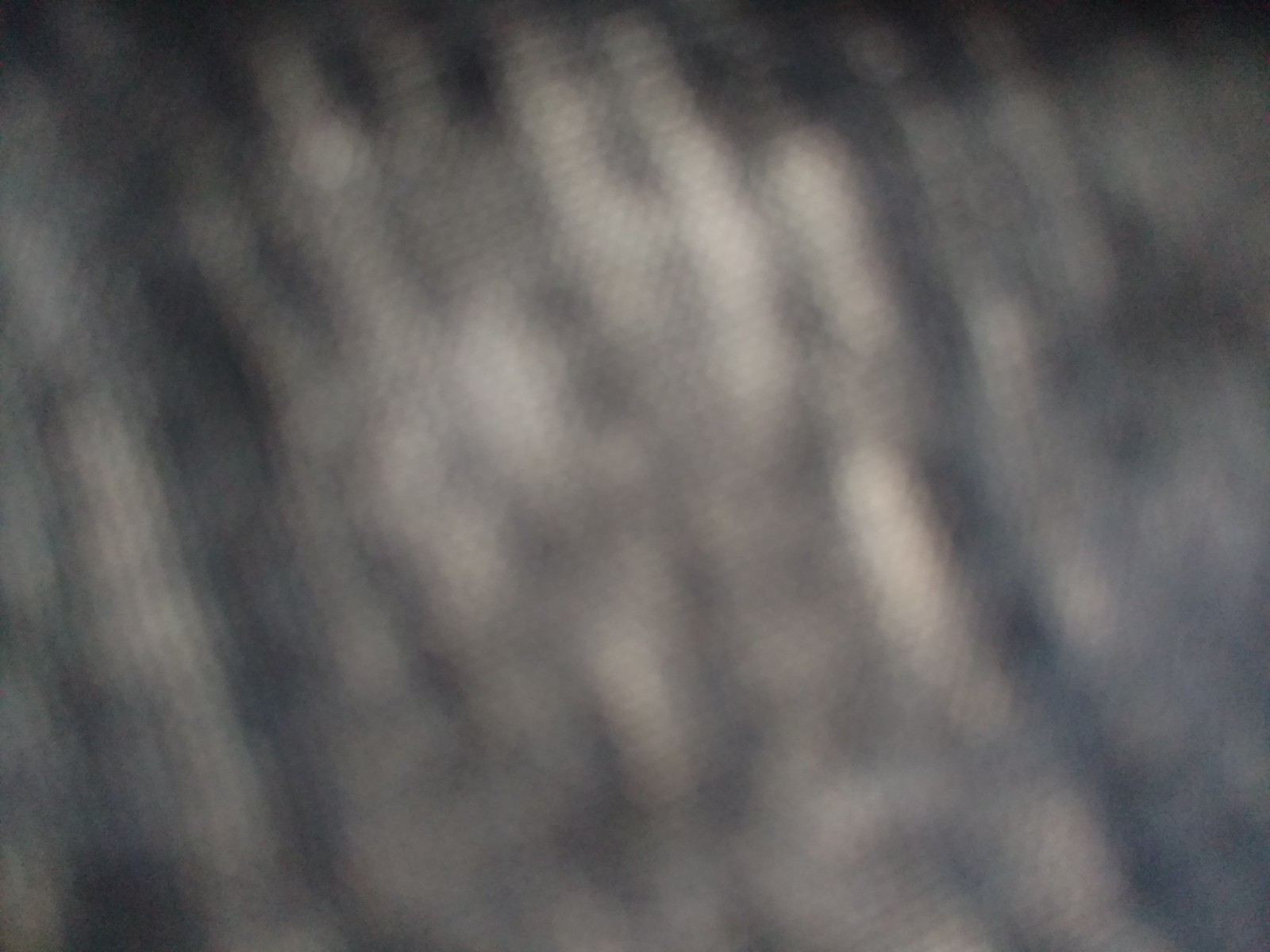A highly abstract and impressionistic black and white image predominates the frame, characterized by an array of blurred forms and opaque textures. The composition is heavily dominated by a grayish-blue color palette, interspersed with random white splotches that subtly punctuate the scene. The image lacks discernible objects, maintaining an enigmatic and somewhat ethereal quality. Darker patches of grayish-blue add depth and variation, contributing to the overall sense of obscurity and amorphousness. The lack of sharp lines or recognizable shapes evokes a mysterious and contemplative atmosphere, inviting the viewer to imagine forms and narratives within the indistinct blur.